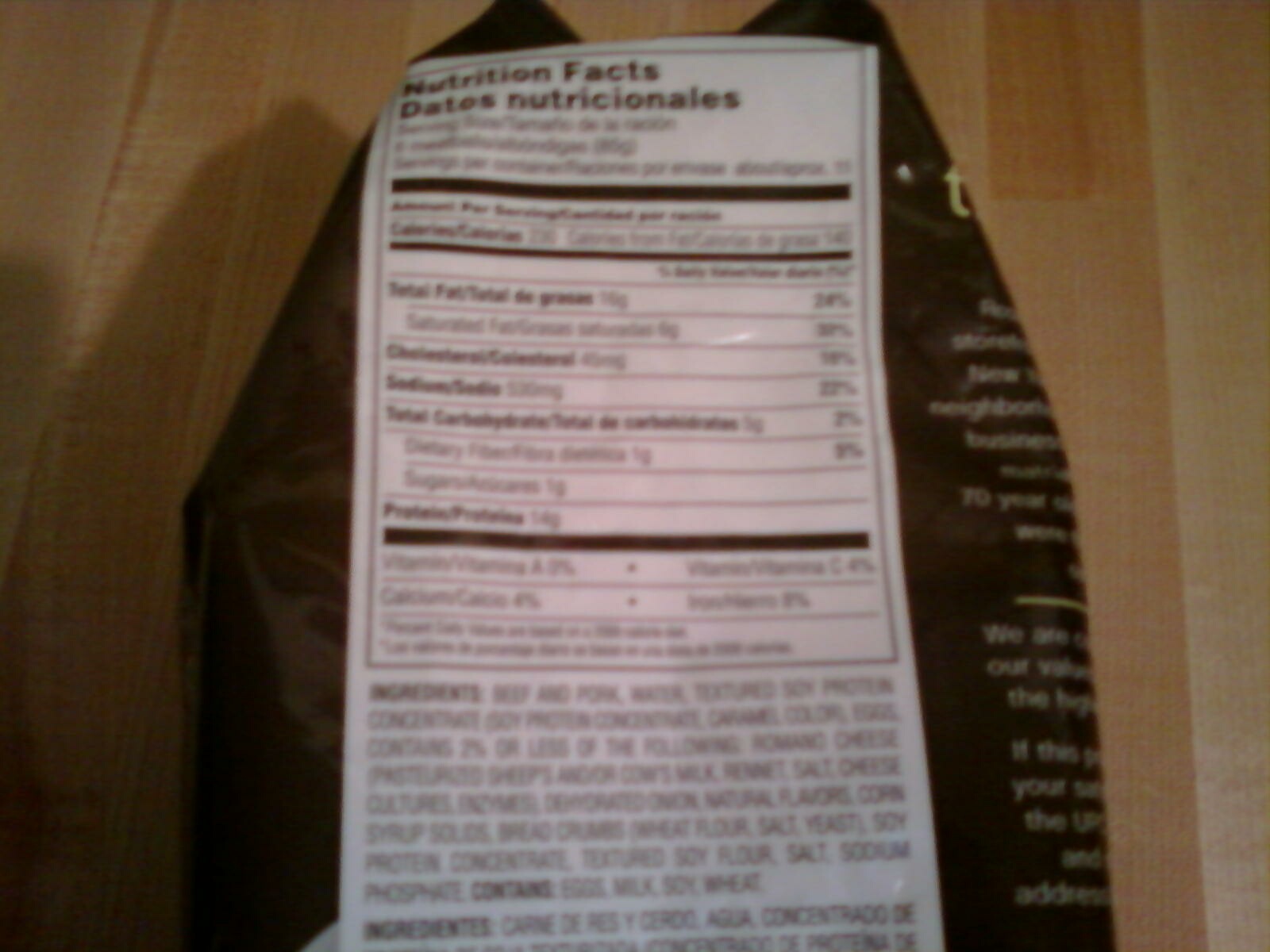The image depicts a bulging, dark brown, or black snack packaging, resembling a potato chip bag, resting on a light-colored wooden countertop with vertically arranged slats. The visible side of the bag prominently displays a blurry white nutritional facts panel and ingredients list, written in both English and Spanish. The detailed label, which includes warnings about allergens such as eggs, milk, soy, and wheat, occupies a significant portion of the blurry bag's side. The packaging's somewhat square shape and the side panel's unreadable small text add to the overall indistinct appearance of the photograph.